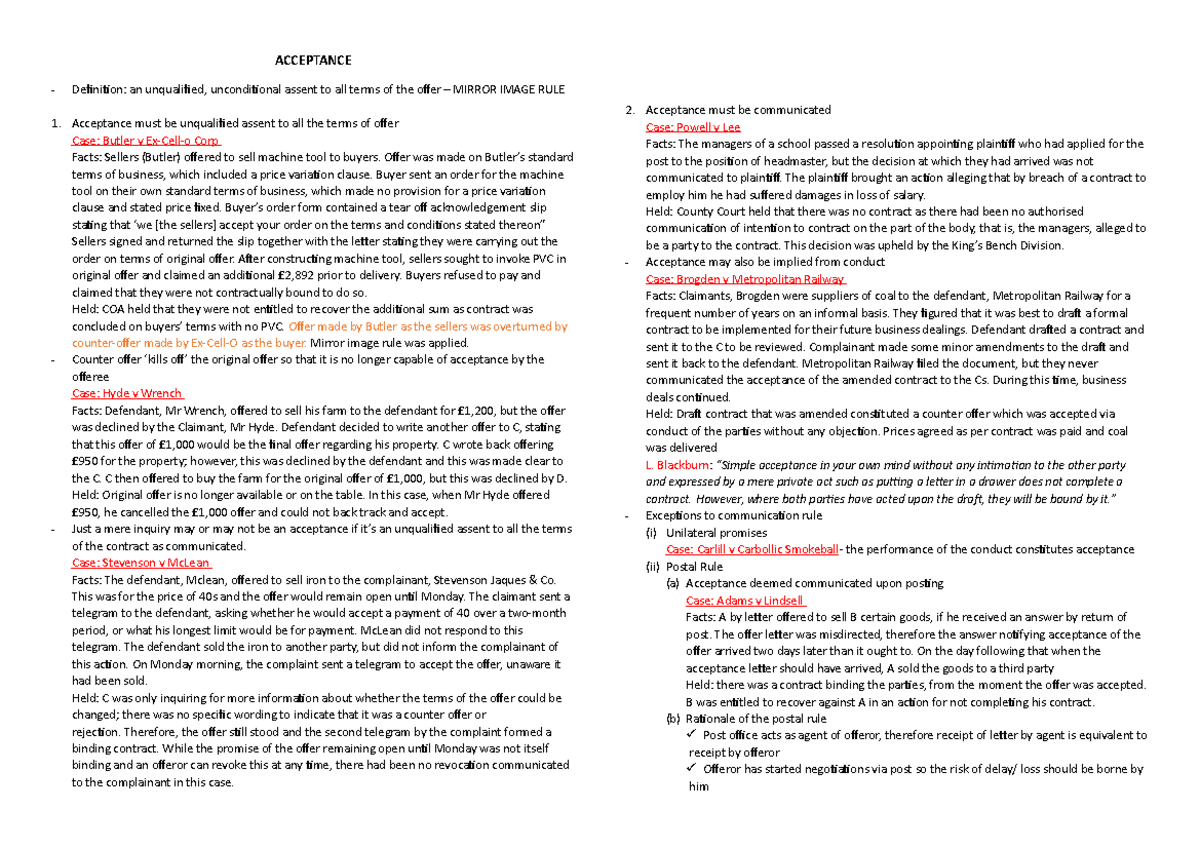**Detailed Caption:**

The screenshot displays two lengthy paragraphs focused on the legal concept of acceptance in contract law. On the left side, labeled "1. Acceptance," it is defined as "an unqualified, unconditional assent to all terms of the offer," adhering to the mirror image rule. The first page highlights three sections in red, each referencing specific cases: "Case Butler vs. Excello Corp.," "Case Hyde vs. Ranch," and "Case Stevenson vs. McLean."

The second page is marked "2. Acceptance Must Be Communicated," listing several pertinent cases such as "Case Powell vs. Lee," "Case Brogdon vs. Metropolitan Railway," "Blackburn," "Case Carroll vs. Carbolic Smokeball," and "Case Adams vs. Lincell." Underneath the Blackburn case, the text is further divided into explanatory sections: "(I) Unilateral Promises" and "(II) Postal Rule." The Postal Rule section includes subpoints "(A) Acceptance Deemed Communicated Upon Posting" and "(B) Rationale of the Postal Rule," with two check marks noted below subpoint B.